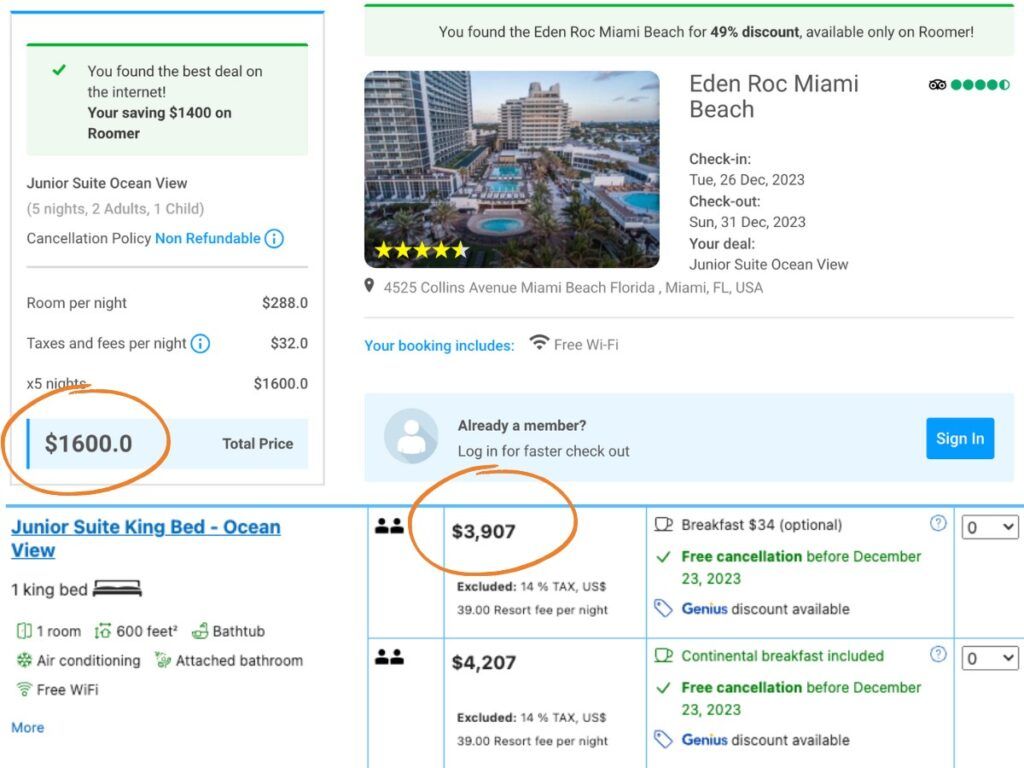The photograph features the luxurious Eden Rock Miami Beach Hotel, a prominent high-rise building renowned for its opulent accommodation and amenities. In the foreground, three distinct swimming pools sparkle under the sun, inviting guests for a refreshing dip. Highlighted by a prestigious 5-star rating, this establishment promises an exceptional experience.

This particular booking is for a Junior Suite with an Ocean View, ensuring a scenic stay with breathtaking vistas. The reservation spans from Tuesday, December 26th, 2023, to Sunday, December 31st, 2023. Valued at just over $5,000, this comprehensive package includes essential amenities such as free Wi-Fi. The convenience of complimentary internet access adds significant value, making this splendid getaway both luxurious and connected.